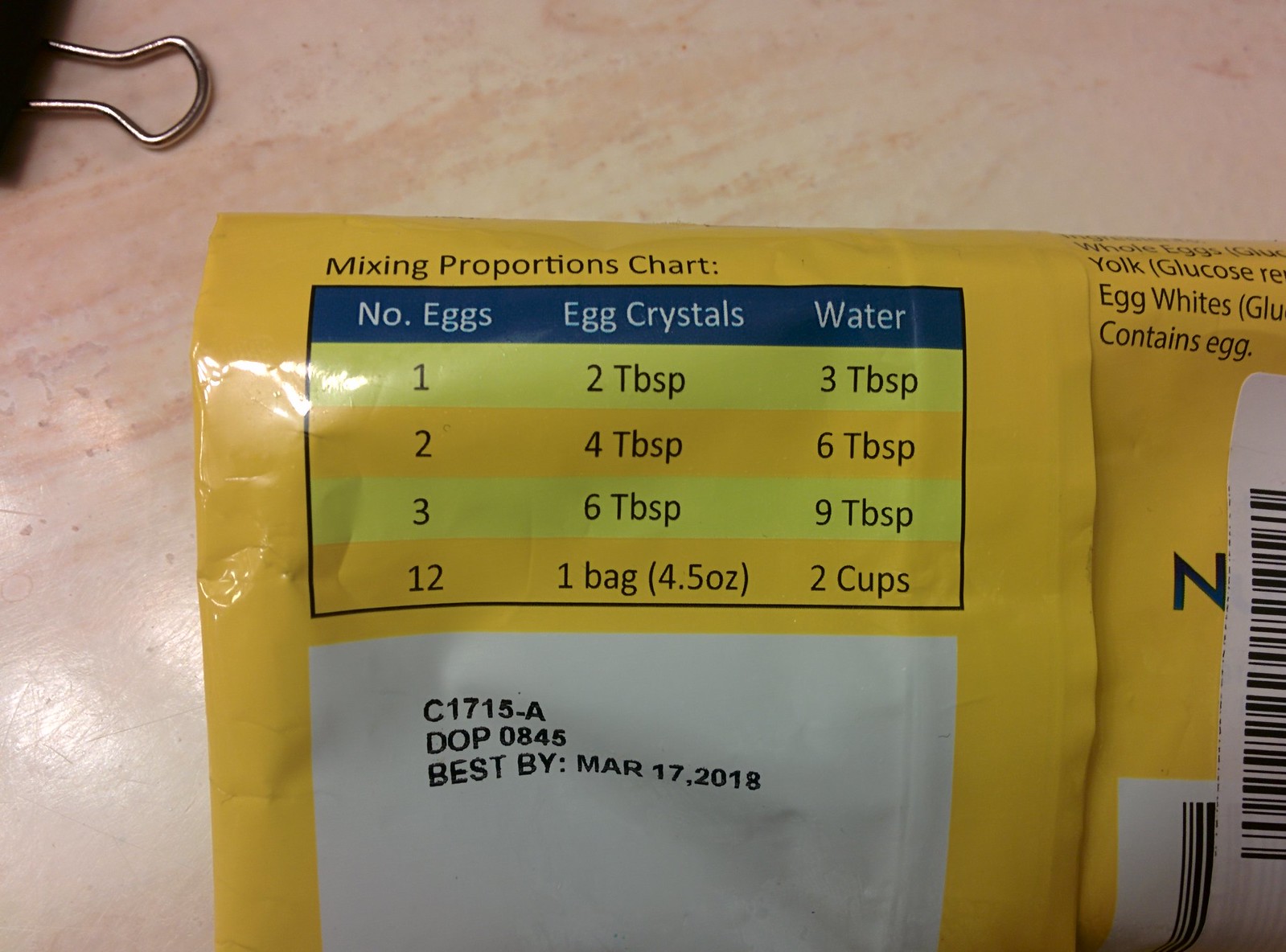This colored photograph depicts the back of a yellow food packaging resting on a marble-like surface with a pale pinkish hue. The focal point on the upper left is a "Mixing Proportions Chart" written in white against the yellow background, providing detailed measurements: one egg corresponds to two tablespoons of egg crystals and three tablespoons of water; two eggs to four tablespoons of egg crystals and six tablespoons of water; three eggs to six tablespoons of egg crystals and nine tablespoons of water; and twelve eggs (equivalent to one bag, which is 4.5 ounces) require two cups of water. Below this chart, a blue rectangle with white text enumerates these proportions. Directly beneath it is a white rectangle displaying a "Best By" date of March 17th, 2018, and some black text indicating the lot number. Towards the upper right, the packaging reveals part of the ingredient list, including egg whites, whole eggs, yolk, glucose, and an indication that it contains eggs. There are two barcodes visible: a smaller one at the lower right corner and a taller, thinner one overlaid on it, partially obscuring additional text. A metallic clip with a black corner is visible at the top of the package, while light reflects off the edge, illuminating parts of the packaging. The visible portion of the package implies continuation, suggesting the existence of more content extending to the right side.